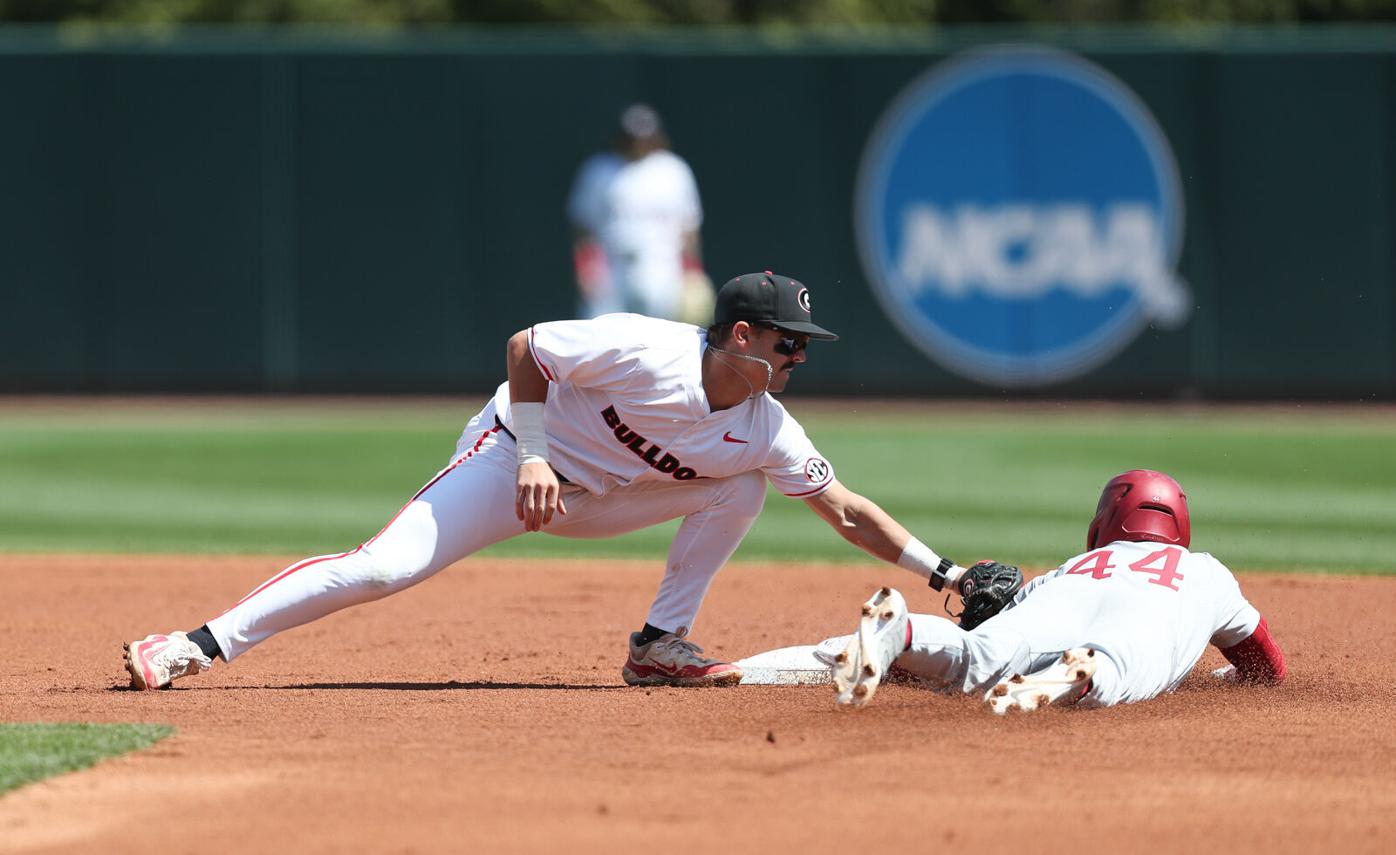The image captures an intense moment during a baseball game, likely at the collegiate level, featuring a close-up of two players in action on the diamond. The player on the right, wearing a red helmet, red sleeves, and a white uniform with the number 44 on the back, is sprawled on the ground near home plate. The player on the left, identified by his black "Bulldog" cap and Nike-branded shirt, is leaning down with his black mitt touching the player on the ground, suggesting he is tagging him out. Both players are wearing cleats and their uniforms feature red and black accents. The background shows a baseball field with a blurred-outfielder and greenery, and a prominently displayed blue circular logo with "NCAA" written in white.